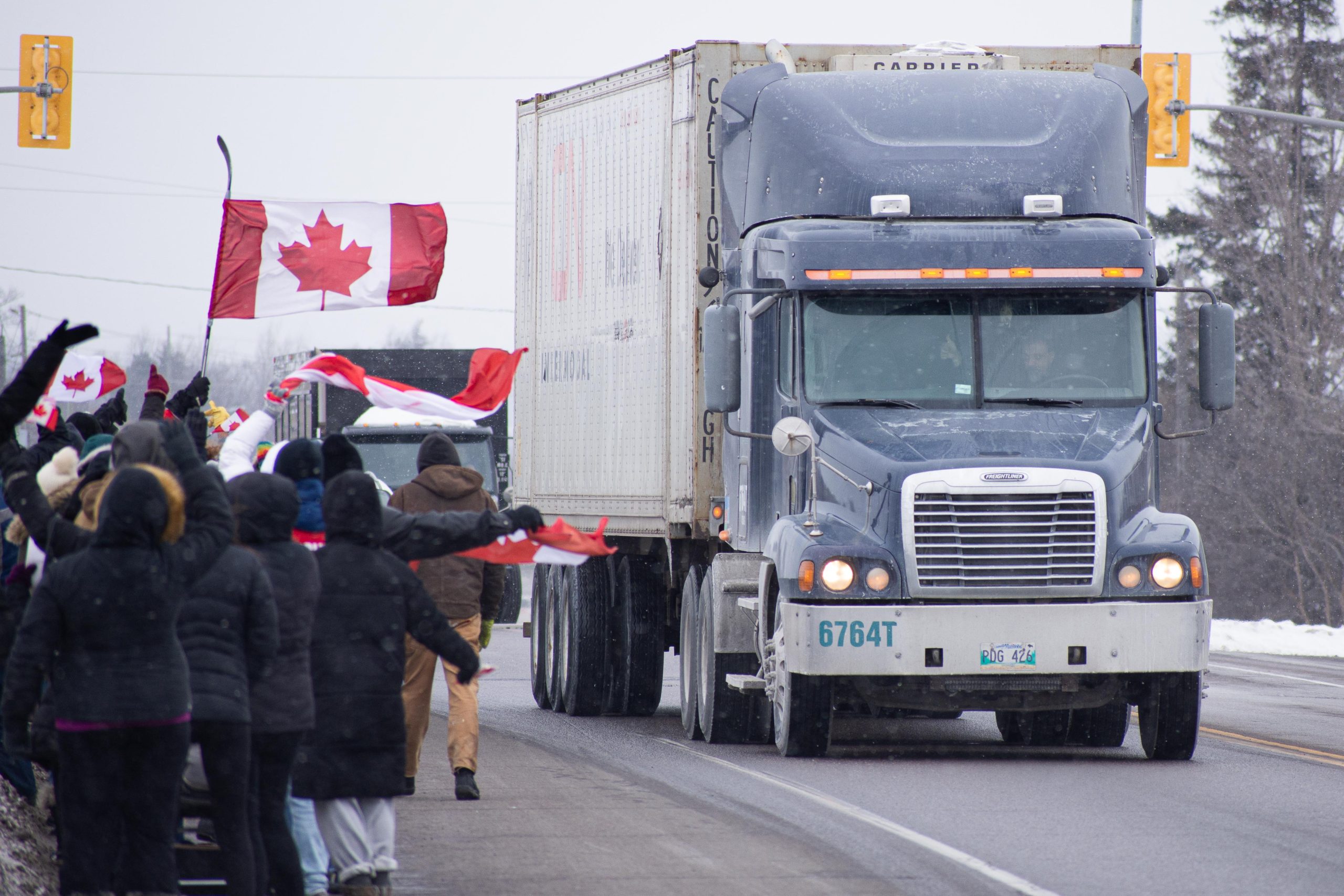In this winter scene set on a snow-dusted Canadian highway, a blue semi-truck with a white trailer takes center stage as it drives down a two-lane road. The truck, marked with the number 67614 on its front bumper, is accompanied by another dark blue box truck trailing behind. The surroundings are stark, with leafless trees and what appears to be stoplights in the background, conveying a chilly, snowy atmosphere.

On the left side of the image, a crowd of 15 to 20 warmly-dressed people stand on the shoulder of the road, waving vibrant red and white Canadian flags adorned with the iconic red maple leaf. The people, clad in winter coats, gloves, and hats, appear to be either celebrating or supporting the truckers as they pass by. The truck driver reciprocates the crowd's enthusiasm with a thumbs-up gesture, adding a personal touch to the spirited roadside gathering.